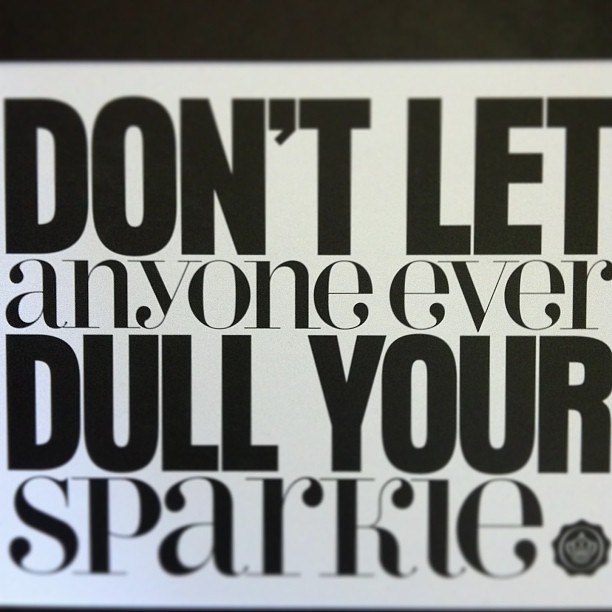The image is a close-up of an inspirational saying, prominently displaying the text "Don't let anyone ever dull your sparkle" in a mix of large black block letters and smaller lowercase lettering. The background is a pale blue with a black rectangular bar running across the top, slightly out of focus. The text is presented in a sequence: at the top, "don't let" in large block letters; below, "anyone ever" in smaller, sharper lowercase letters; followed by "dull your" again in large block letters; and finally, the word "sparkle" in smaller, slightly out-of-focus lowercase letters. In the lower right corner of the image, there's a small insignia within a dark circle, featuring a scalloped edge. This insignia contains a slightly blurry gold emblem that resembles either a crowned chess piece or a monkey's face, making it difficult to distinguish clearly.